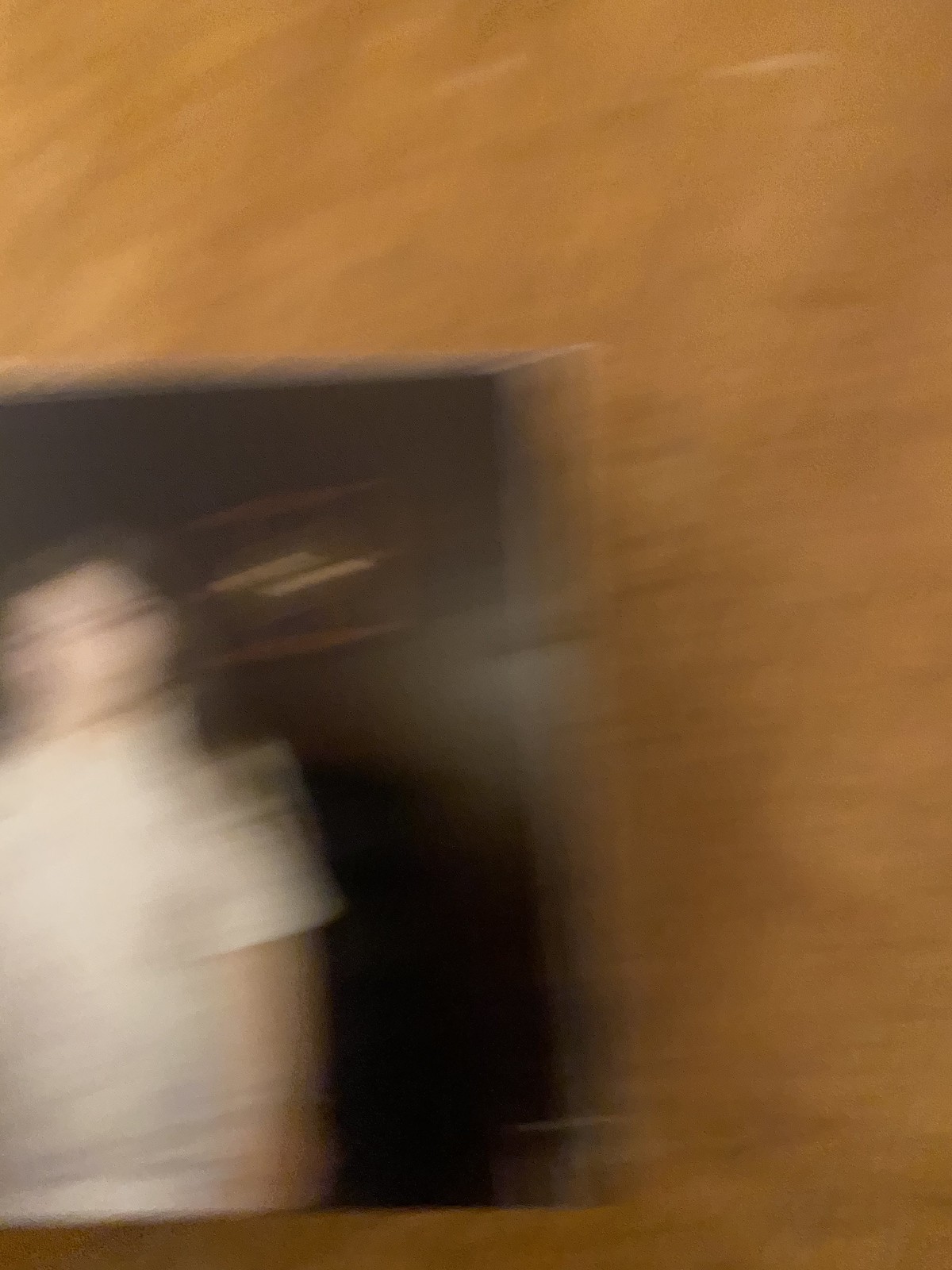This is a highly blurred and out-of-focus image, capturing a photograph that is placed on a light brown or darker tan surface, possibly a table. The background of the original photograph is predominantly black, punctuated by a few streaks of light, suggesting movement and resembling stripe-like patterns. The visible portion of the photograph reveals a person wearing a white short-sleeved shirt. They have fair skin and dark hair, though the facial features are indistinguishable due to the lack of focus. This photograph might be a frame from a rapidly moving video, which could explain the elongated, stripe-like appearance of the lights in the background.